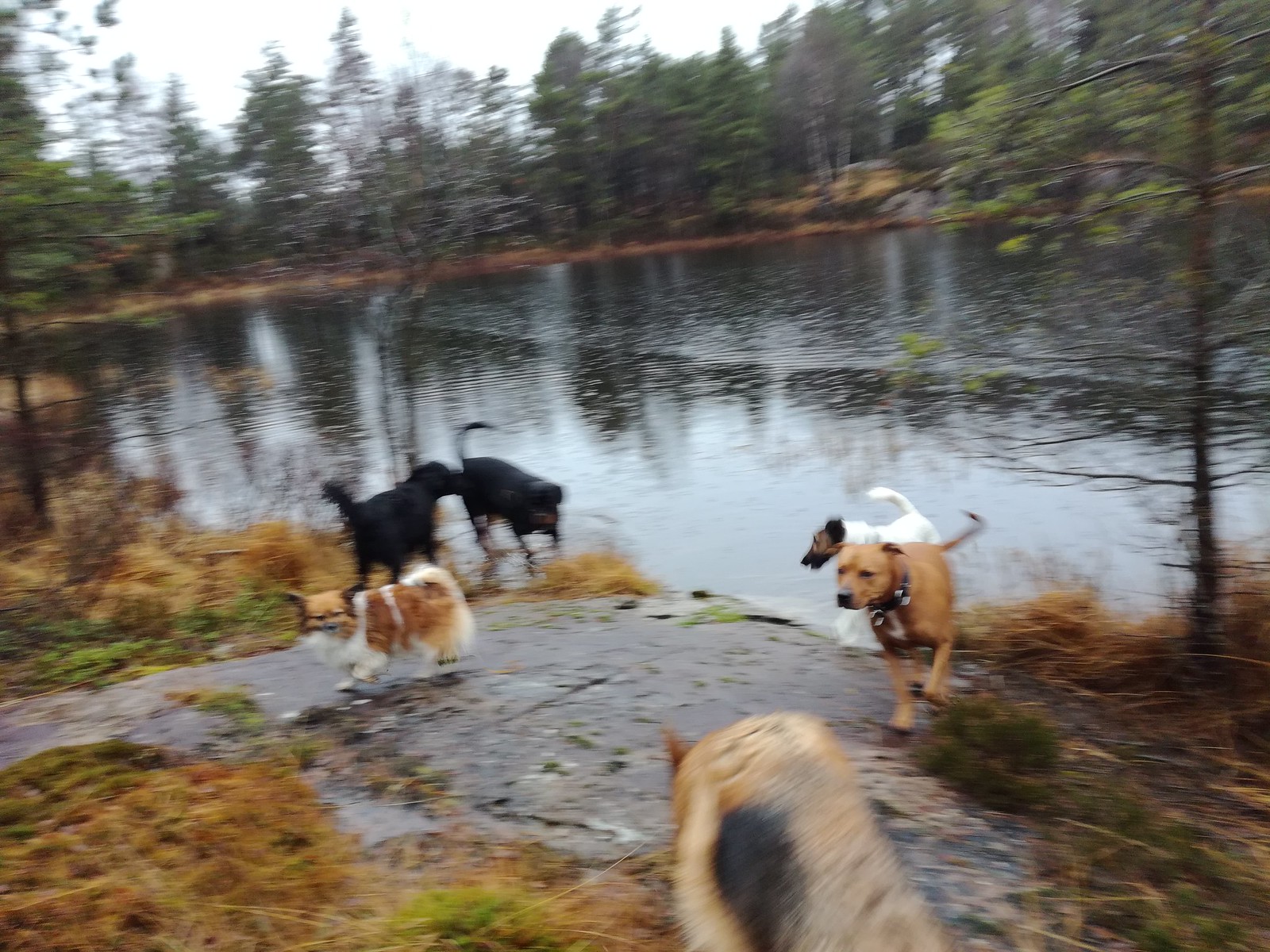This image depicts a dynamic scene near a lake surrounded by lush, green trees. Despite the motion blur, six dogs of various breeds and sizes are clearly visible. In the foreground, there is a small hill with patches of dirt and brown-green grass. On the right, a brown pit bull with a black collar stands amidst the action while a white dog with a brown face is positioned behind it. Two large black dogs are in the background, one of which is wading in the lake. The left side of the image features a small, fluffy brown and white dog with long fur and a distinctive white tail that curls over its back. Additionally, the partial view of a light brown dog with black ears is seen towards the front. The sky appears almost white, contrasting with the vibrant greenery encompassing the serene lake, creating a picturesque backdrop for this gathering of playful canines.